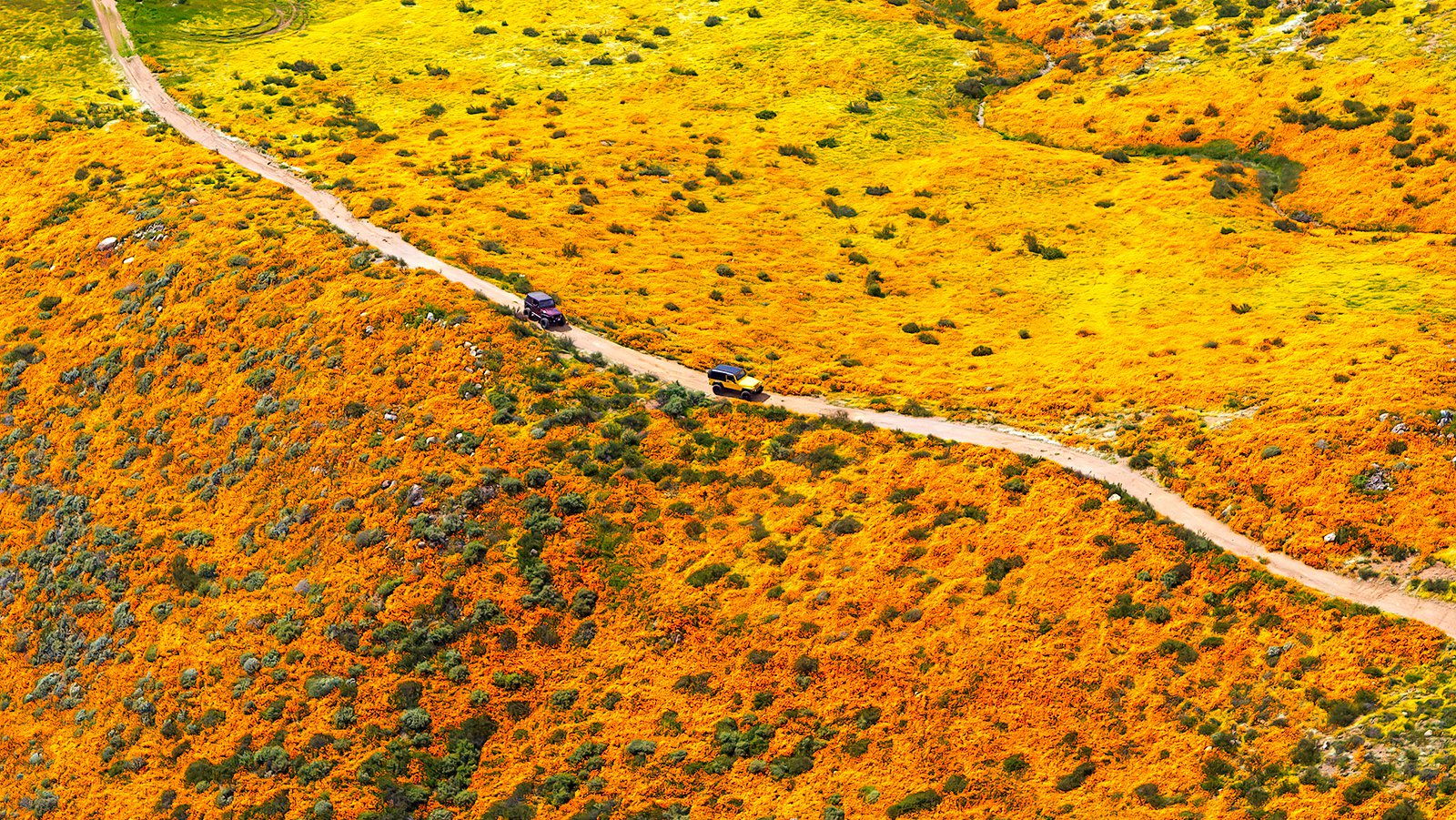This detailed aerial photo captures a sunlit afternoon drive through an expansive desert landscape. A one-lane, light-brown road stretches diagonally from the top left to the bottom right of the frame. Traversing this road are two jeeps, the lead vehicle a vibrant yellow with a black top, followed by a jeep of a purplish hue, also with a black top. The surrounding terrain is a patchwork of orange and yellow hues, interspersed with patches of green. The vegetation primarily consists of low-lying bushes and prickly plants that are scattered irregularly across the desert, indicating the sparse, harsh environment. The ground color varies with shades of orange, green, red, purple, gray, and blue, giving the scene a rich and varied palette. The vast, barren expanse and the solitary vehicles evoke a sense of isolation and adventure in this rugged, open wilderness.